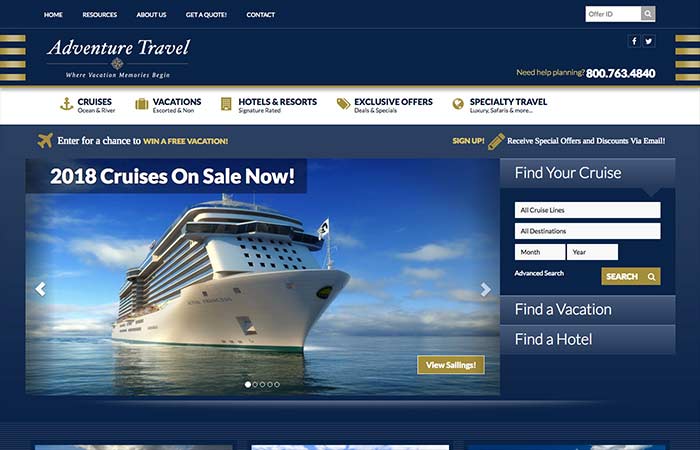The webpage titled "Adventure Travel" prominently features its name in white text at the top left corner. Directly to the right, the name "Blair" appears, also in white. Above these elements is a navigation bar with tabs for Home, Resources, About Us, Get a Quote, and Contact, all set against a dark blue background. 

On the top right, users can access a search button, as well as Facebook and Twitter icons for social media engagement. Below, the contact number "Need help planning? 800-763-4840" is displayed. 

The main content section features a white background with dark blue text and gold icons. The navigation tabs here include: "Cruises (Ocean and River)", "Vacation", "Excursion", "Hotel and Resort", "Signature Road", "Exclusive Offers, Deals and Specials", and "Specialty Travels". 

To entice visitors, a segment on the left announces, "Enter for a chance to win a free vacation," accompanied by an image of a white cruise ship sailing to the left against a backdrop of a blue ocean and a sky with grey clouds. Above the ship, the text "2018 Cruises on sale now" stands out in white, and a gold button below reads "You Sailing".

On the right side of the image is a search menu titled "Find Your Cruise," which allows users to filter options by cruise line, destination, and dates with categories for "All Cruise Lines," "All Destinations," "Month and Year," and an "Advanced Search" option. Another gold button labeled "Search" is positioned at the bottom.

Finally, at the bottom right, two blue buttons offer further actions with "Find a Vacation" and "Find a Hotel."